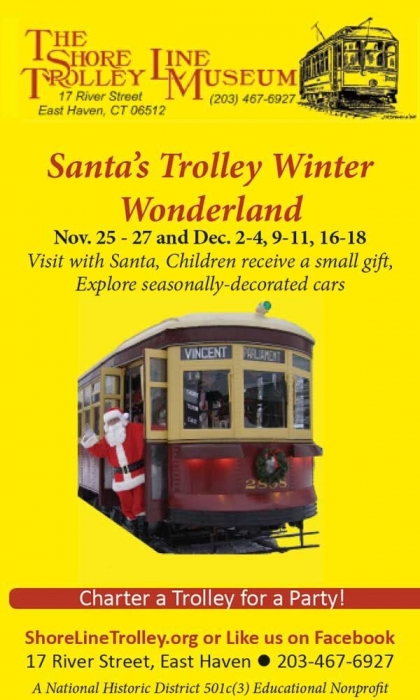The advertisement poster is a bright, cheerful yellow, designed in a long, portrait layout. At the top, a hand-drawn black trolley is displayed, followed by the title "The Shoreline Trolley Museum" in bold red letters. Directly below, in black text, is the address: "17 River Street, East Haven, Connecticut, 06512," and the phone number: "203-467-6927." A notable addition is the mention that it is a "National Historic District 501(C)(3) Educational Nonprofit."

In red text, "Santa's Trolley Winter Wonderland" is prominently advertised. The event is scheduled for November 25-27 and December 2-4, 9-11, and 16-18, with details in black text highlighting activities such as "Visit with Santa," where children receive a small gift and explore seasonally decorated cars.

Towards the bottom, there is a colorful photograph of a vibrant red trolley with a Christmas tree at the front, and Santa, donned in his classic red-and-white attire, waving from the open door. Below this image, a red-bordered banner invites people to "Charter a Trolley for a Party," and provides further contact details: "shorelinetrolley.org or like us on Facebook." The bottom of the poster reiterates the address and phone number in black text, ensuring easy accessibility for interested parties.